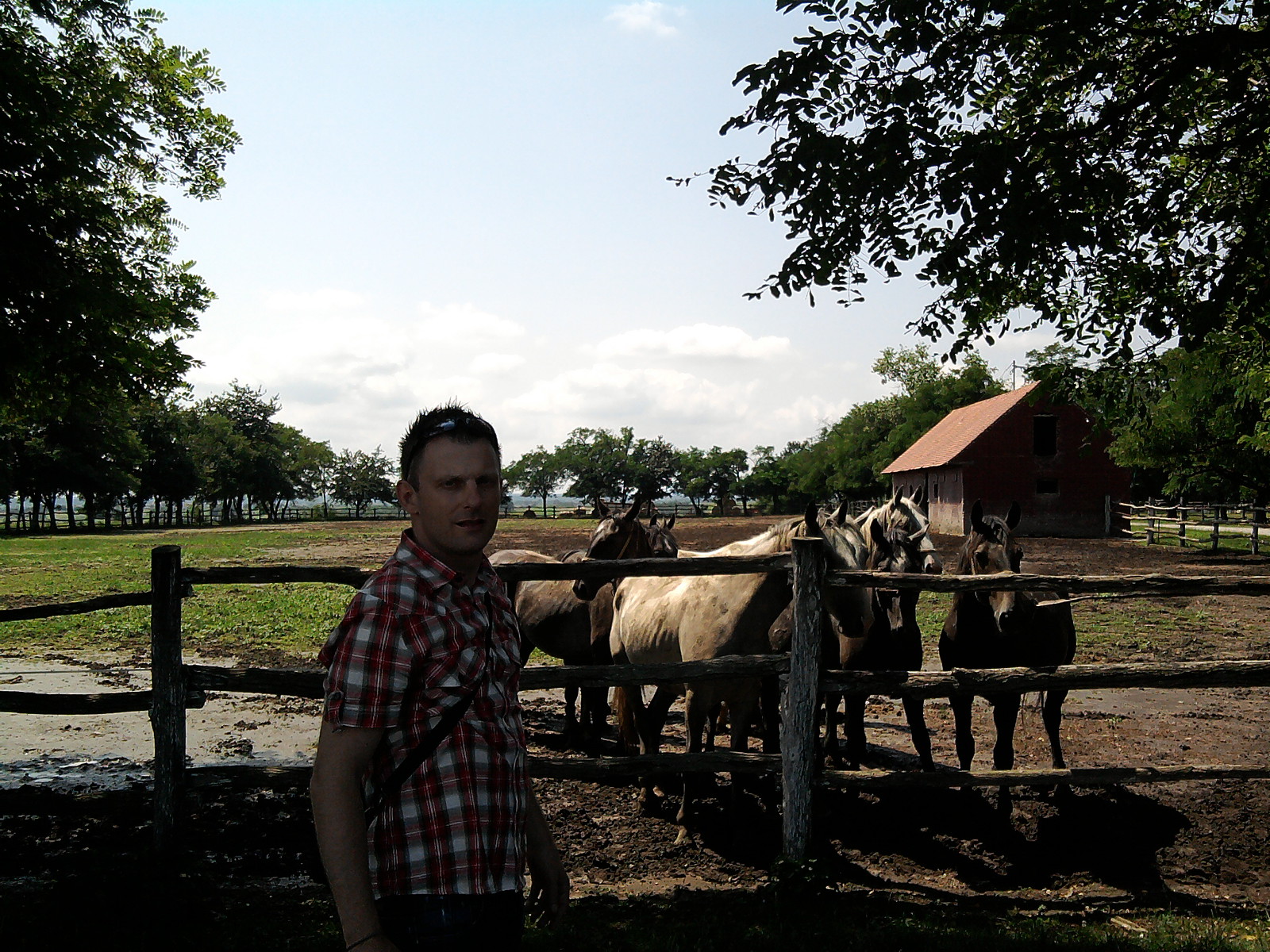In this detailed photograph, a Caucasian man stands in front of a wooden fence, dressed in a red, white, and black plaid shirt and sporting sunglasses on top of his head. He carries a sling bag and showcases a neutral expression. Behind the man, several horses, primarily light brown and dark brown, gather close to the fence—six in total, some adorned with white markings on their manes. The setting extends to a dirt and grass pasture enclosed by lush green trees. A small red barn with an A-frame roof occupies the background, indicating a rustic and serene scene. The sky above is a mix of bright blue and scattered clouds, providing a picturesque backdrop to this tranquil farm setting.